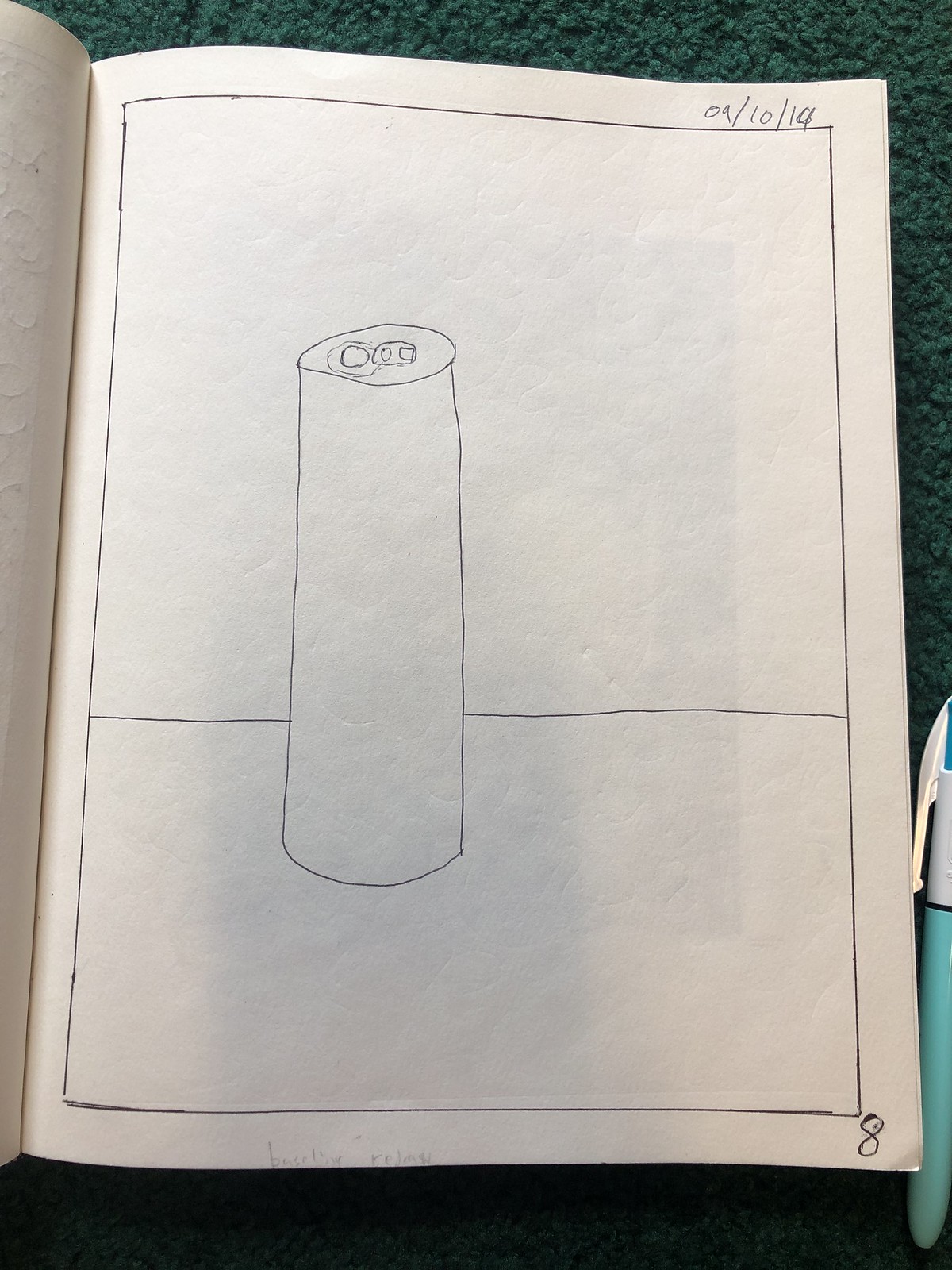This photograph features a simple pencil line drawing displayed within a white sketchbook. The sketchbook lies open, filling the majority of the frame with its vertical rectangular page. A slight curve of the opposite page is visible on the left side. The book rests on dark green carpet, which appears in thin strips around the upper, lower, and right edges of the frame. 

In the lower right corner, a light blue and white pen or mechanical pencil is seen parallel to the open page. The drawing itself is a rudimentary black line drawing featuring a rectangular border. Within this border, there is a horizontal wall line and a tall, narrow can depicted with a pop tab on top. The lines throughout the drawing are fairly wobbly and lack parallelism, indicating the creator is not an experienced artist. 

The artwork is dated "09/10/19" in the upper right corner, and the number "8" is inscribed in the lower right corner of the page.